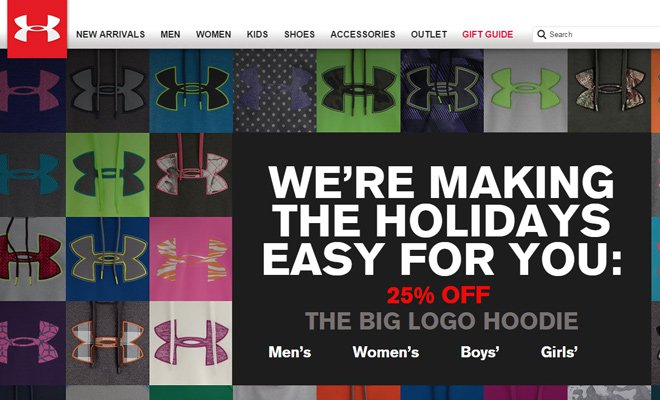The image depicts an Under Armour launch page, designed as a webpage viewed on a computer. At the top of the page, there is a prominent white menu bar. On the left side of this bar, a red box features the distinctive Under Armour ("UA") logo, which consists of two intersecting half-circles forming an abstract "UA" shape. The menu items listed in black text include "New Arrivals," "Men," "Women," "Kids," "Shoes," "Accessories," "Outlet," and "Gift Guide," with "Gift Guide" highlighted in red.

To the right of the menu, there is a search bar with the placeholder text "Search" displayed in gray and an adjacent magnifying glass icon to its left.

Below this menu bar, the page showcases numerous Under Armour logos in various colors and backgrounds, including shades of pink, gray, black, green, camo patterns, tiger camo, red, and even a plaid design. Most of these backgrounds are solid colors, except for one that features black and white polka dots, and others predominantly appear in tones of gray, pink, or purple.

Occupying the bottom third of the image is a black box. Inside this box, there is white text stating, "We're making the holidays easy for you." Below this, in striking red text, it reads, "25% off.” Further information in gray text advertises "the big logo hoodie," and this is followed by a list in white text indicating the offer is available for "Men's," "Women's," "Boys'," and "Girls'."